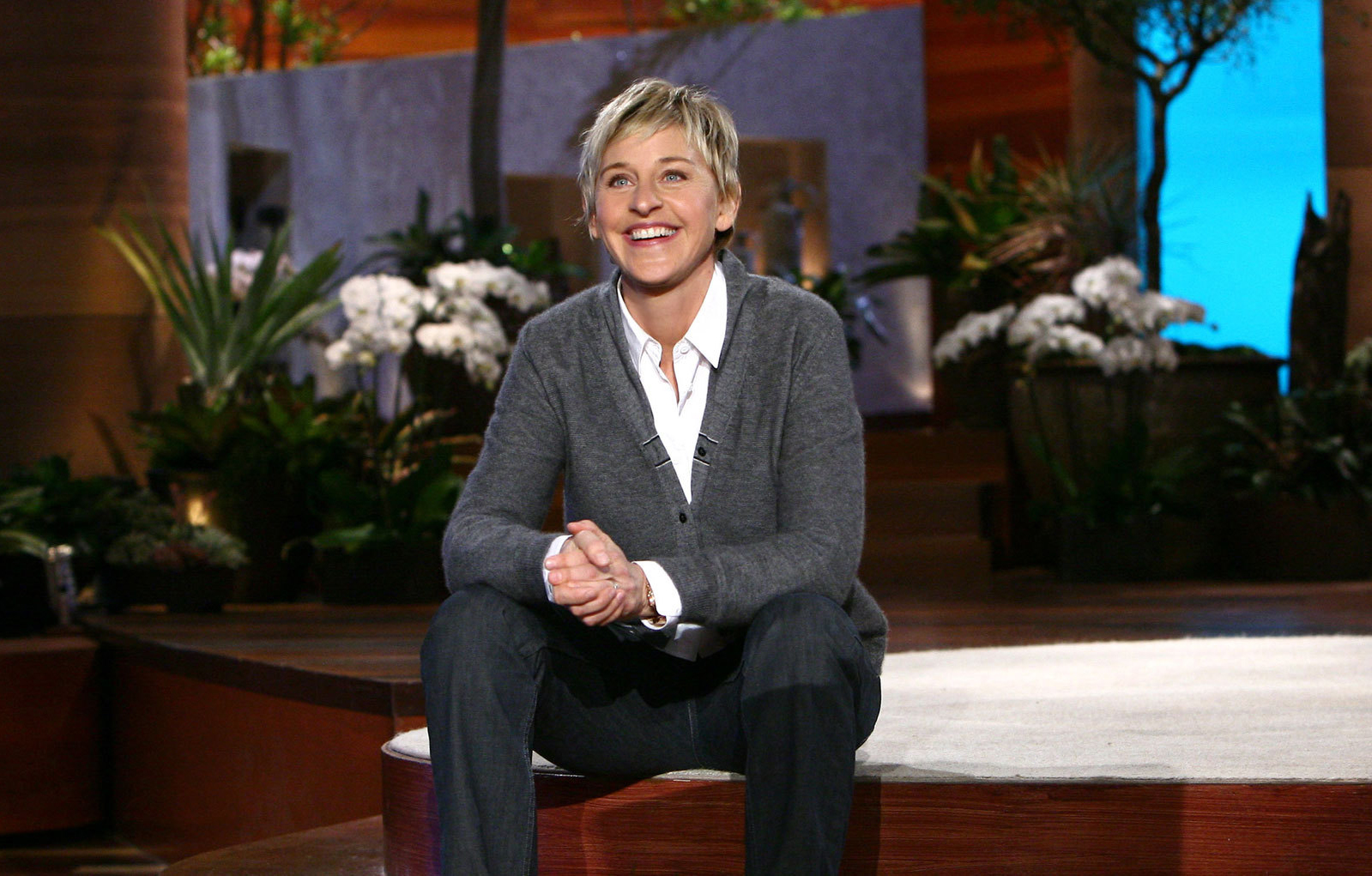The photo features television host Ellen DeGeneres sitting on the edge of a circular platform, which appears to be part of her studio stage. Ellen, with her short, boyish-style blonde hair, is smiling broadly, looking both confident and welcoming. She is dressed in a dark gray cardigan with buttons over a white collared shirt, paired with dark navy blue pants. Her hands are clasped in front of her as she sits on the cherry wood-colored platform. The backdrop consists of an array of indoor plants, including green leaves and white flowers in pots and planters, set against a light bluish-gray background with additional cherry wood elements. The lush greenery and Ellen's warm expression create an inviting and relaxed atmosphere in the image.